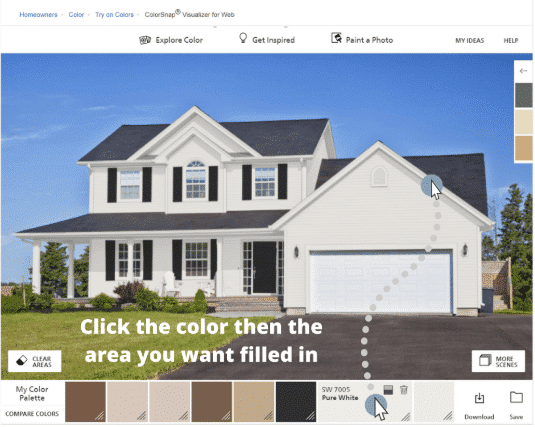The image depicts a large, white house with gray roofs, featuring six windows and a white garage door. The house is set against a backdrop of a clear blue sky and lush green grass. Text on the house reads, "Click the color, then the area you want filled in." Beneath the house, there is a color palette labeled "My Color Palette," offering various color options for user selection. Over the house, a banner displays the text: "Homeowners, Color Try-On, ColorSnap Visualizer for Web." This suggests that the image is part of a website designed for users to customize and visualize different color schemes for their homes. Additionally, the image includes two blue dots connected by a line of smaller blue polka dots.